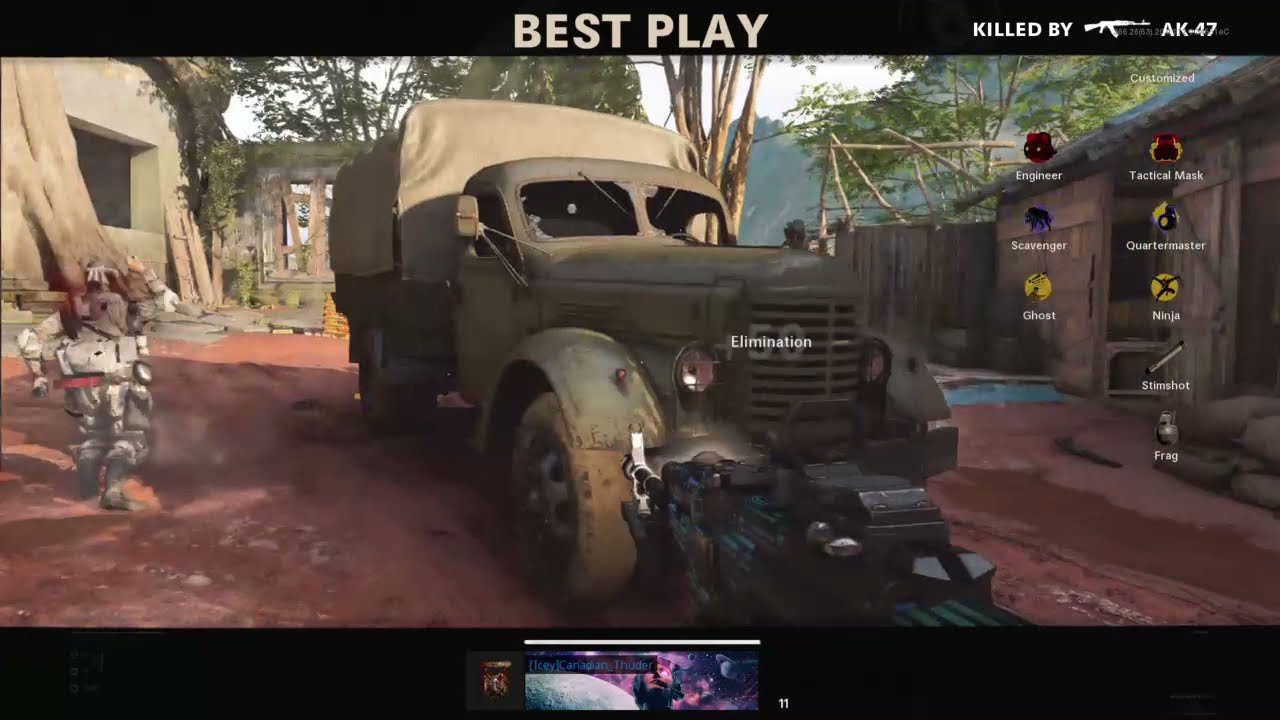In this image, we see a screenshot from a video game. The screen has black header and footer bars, with the header displaying "Best Play" in bold, off-white letters, and "Killed by AK-47" along with an outline of an AK-47 in the upper right corner. In the center of the main image, there's a large, green army truck with smashed windshields and a green cover over its back, concealing its contents. An unusual, large gun is aimed towards the truck from the left side of the screen. A soldier, appearing to be a human-robot hybrid, is running away from the truck, dressed in an all-white and gray army outfit.

In the background, there's a detailed jungle camp setting with a reddish-brown dirt ground. To the left of the truck, there’s a house that’s green and tan in color. Further right, there’s a brown fence, a small brown building, some green army bags, and trees extending into a mountainous area. The right side of the screen features a vertical list of customization options in white letters, including "Engineer," "Tactical Mask," "Scavenger," "Quartermaster," "Ghost," "Ninja," "Stim Shot," and "Frag."

At the bottom center of the footer, there’s a small block depicting a scene of outer space with a planet and possibly another planet in blue and purple hues, though it’s only faintly visible. This image combines an intense jungle warfare scene with a tactical overlay typical of a first-person shooter video game.